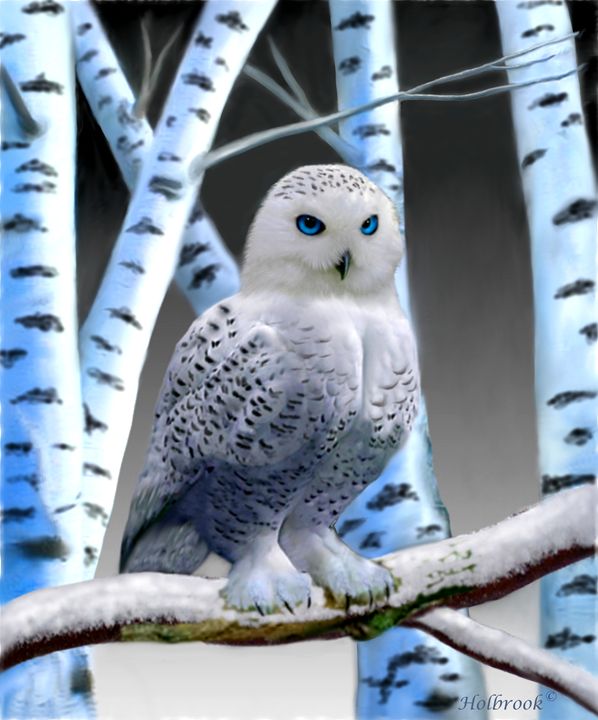This highly detailed image, likely a realistic painting or computer-generated art, depicts a captivating snowy owl perched on a snow-covered branch. The owl, positioned prominently in the center, has arresting bright blue eyes, a small black beak, and white feathers adorned with scattered black markings across its body, wings, and head. The background features five slender birch trees with white trunks and black spots, set against a gradient that transitions from black at the top to white or gray at the bottom. The tree branches, some horizontally aligned and others jutting out, are similarly marked and seem to glow, possibly reflecting the snowy setting. The owl's focused gaze is directed slightly to the right. In the bottom right-hand corner, the text "Holbrook" is visible, suggesting a copyright, and adding to the polished, possibly processed, quality of the artwork.